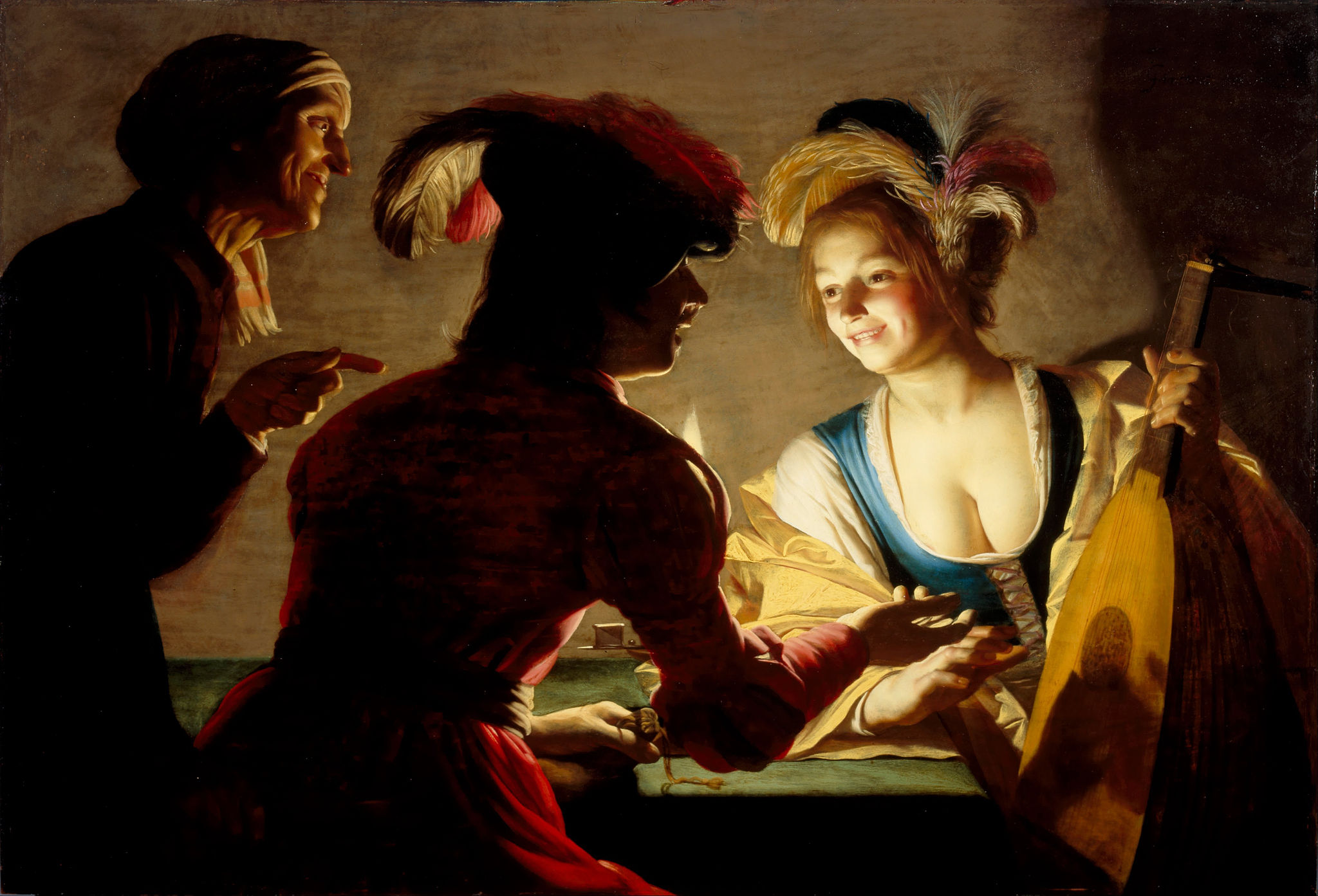This detailed digital artwork, reminiscent of a photorealistic oil painting, depicts a historical scene featuring a young, attractive woman with a fair complexion and red hair adorned with a variety of fluffy feathers in beige, black, gray, and red. She is sitting at a candlelit table, which casts a warm glow on her smiling face and the low-cut neckline of her old-fashioned attire. The young woman, possibly in a tight corset, holds a vintage string instrument, hinting at a musical theme.

Across from her, in the shadows, sit two older individuals - a man and a woman. The man, viewed in profile, is dressed in a red coat with elaborate puffy shoulders and elbows, and has large black and red feathers in his cap. He is gesturing towards the instrument, suggesting a negotiation or haggle. The older woman, also in shadow, stands on the left side, pointing and grinning, giving an air of oversight or instruction. The scene conveys a sense of 1700s or earlier period, accentuated by their old-fashioned attire and the overall sophistication of the composition. The table, draped with a green tablecloth, anchors this engaging tableau of interaction, possibly over the exchange or sale of the musical instrument.